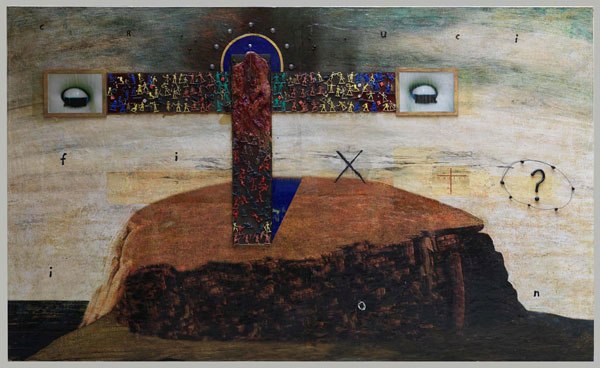The abstract painting appears to depict a surrealist mixed-media scene set against a multicolored background blending whites, grays, blues, oranges, and greens, with subtle hints of a plateau or mountainous landscape under a sky mixed with yellows and blues. Dominating the center of the composition is a brown tree trunk, from which extends a T-shaped cross made of wood; the horizontal beam is wider than the vertical plank. The cross is visually distinct, adorned with a variety of elements, including a white section with two gray tips in the middle, and tiny army men studded throughout. Above the top of the vertical plank, a halo is clearly visible.

To the right and left of the cross beam are closed eyes with eyelashes. Nearby, randomly dispersed throughout the piece, are symbols such as an "X," a question mark encircled by dots situated towards the right, and random letters including F, J, C, R, and U. Additionally, there is a dark brown oval near the base of the trunk that appears to emerge from a more textured or layered base. The question mark encircled with dots is one of the few readable texts, lending an element of mystery to the artwork. The blend of various media and textures, including what appears to be stickers or glued-on pieces, adds to the depth and intrigue of this detailed, enigmatic creation.